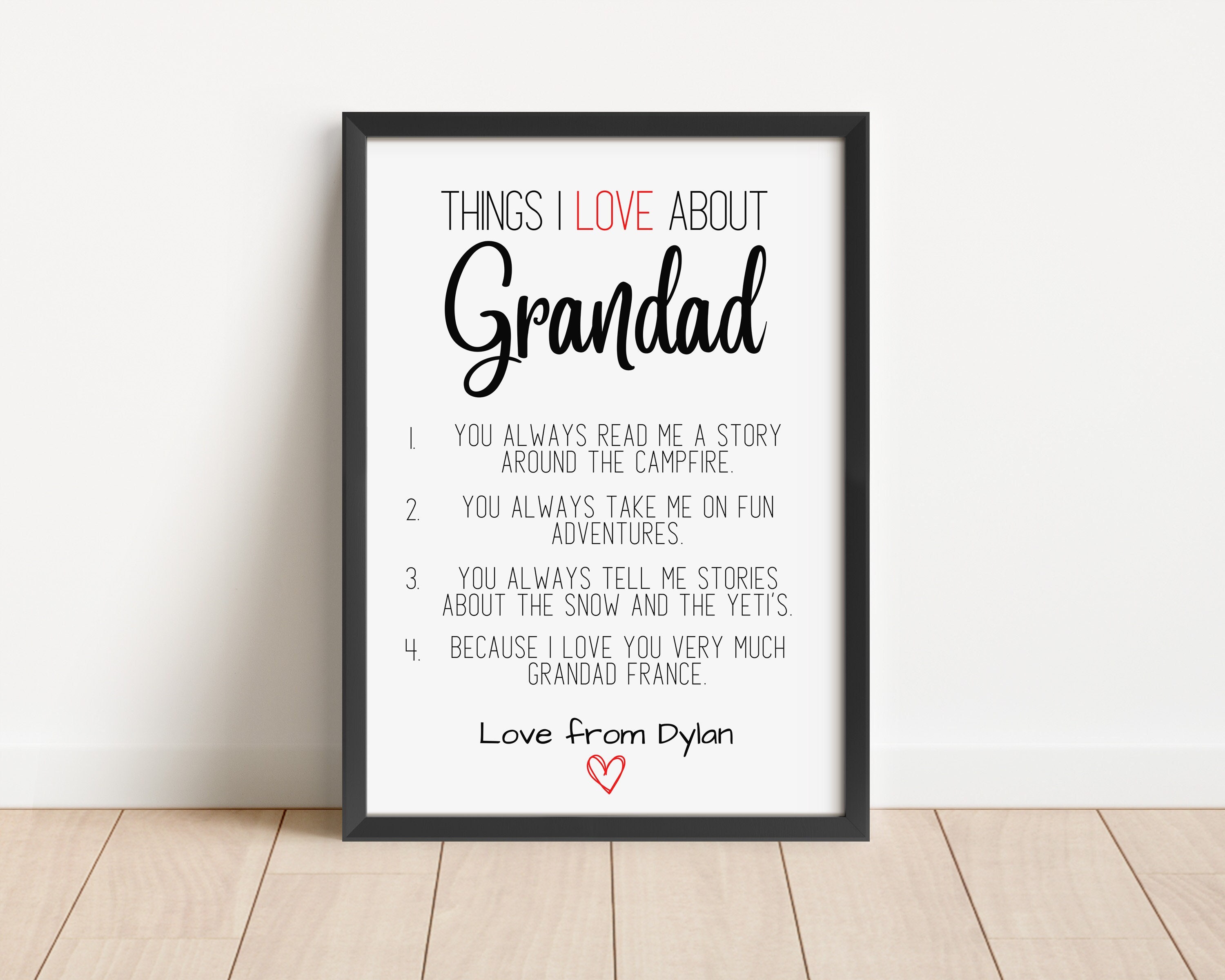The image features a neatly framed decoration leaning against a pristine white wall with light wooden floors beneath. The black frame surrounds a white canvas featuring predominantly black text with pops of red. At the top, in thin, condensed black text, are the words "THINGS I LOVE ABOUT," with "LOVE" highlighted in red. Below this, in large, bold cursive, the word "Granddad" is prominently displayed.

The canvas lists four endearing bullet points in small, condensed thin black text: 
1. You always read me a story around the campfire.
2. You always take me on fun adventures.
3. You always tell me stories about the snow and the Yetis.
4. Because I love you very much, Granddad France.

At the bottom, in a black handwritten-style font, it says "Love from Dylan," accompanied by a cute red-outlined heart. This heartfelt and charming keepsake appears ready to be a cherished gift, perfect for expressing love and appreciation to a grandfather.